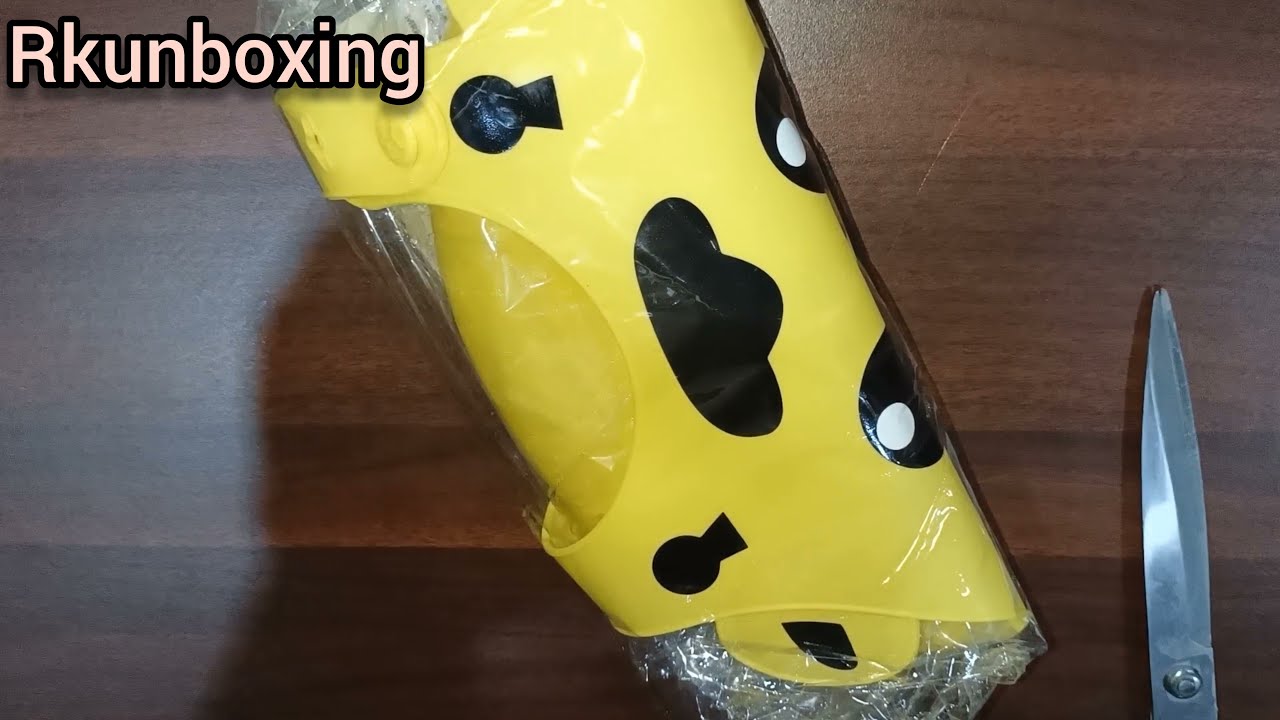The photograph captures a yellow, cartoonish head of a giraffe, made of soft rubber or plastic, which appears to be deflated and intricately folded within a piece of clear plastic wrap. This wrapped item is diagonally positioned from the top left to the bottom right on a dark, faux wood table. In the top left corner of the image, bold text reads "R-K-U-N-B-O-X-I-N-G," with a black outline. The bottom right corner features the shiny silver blades of a pair of scissors, held together by a small bolt. The table also exhibits subtle details like a visible scratch running upward from the lower part of the image to the right and a shadow on the mid-left side, next to the glare of a light source.